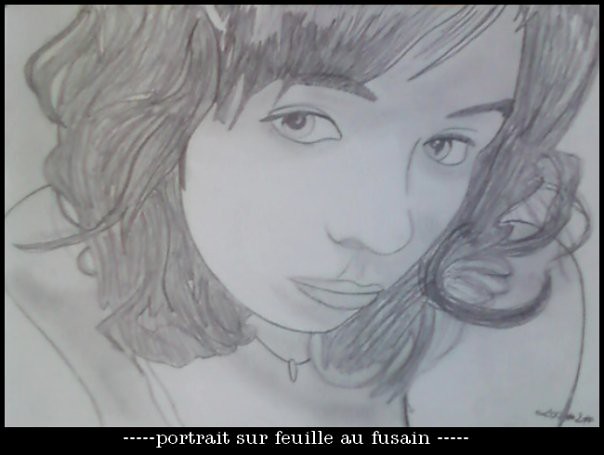The image is a detailed black and white pencil drawing of a woman facing forward with her head slightly cocked to the right. The woman has shoulder-length, wavy hair with bangs that partially cover her eyebrows and wisps of hair going in different directions. Her expressive eyes, which appear sad and slightly averted to the left, convey a poignant emotion. She has prominent round features, including pouty lips and a defined nose. The drawing also features a necklace, possibly a single strand with a pendant resembling a tooth, resting around her neck. Below the woman's upper body, which includes visible shoulders and the collar of a shirt, there is a black border with white text reading "Portrait sur Feuille au Fusain" accompanied by white dots on either side. In the bottom right corner, there is an artist's signature that remains indecipherable. The artwork captures the intricate details of the woman's face and conveys depth with its array of pencil shading techniques.